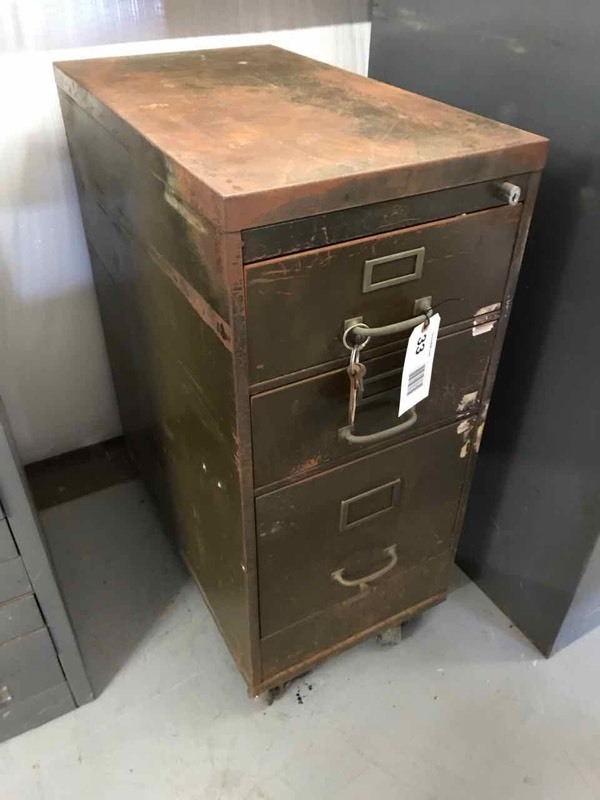The photograph captures a vintage, dark army green metal file cabinet that appears to date back several decades, possibly from the 1920s. The cabinet, heavily worn and rusted, exhibits a significant amount of scuffing and scraping along its edges, revealing exposed metal. The top surface is notably scuffed, displaying rust-colored metal. The cabinet is equipped with caster wheels at the bottom and features three vertically oriented drawers: two shallow drawers on top and a deeper drawer at the bottom, roughly twice the height of the shallow ones.

Each drawer is fitted with a curved, tarnished silver handle and an empty metal label frame, which has also tarnished over time. The top drawer is distinguished by a key ring with a key dangling from it, as well as a white paper tag bearing the number 33 and a barcode. The file cabinet is positioned on a gray floor, up against a white wall, and is flanked on either side by partially visible, more modern-looking gray file cabinets. The surrounding area, as viewed in the photograph, includes a lighter gray cabinet on the left and a darker gray cabinet on the right, both only partially within the frame.